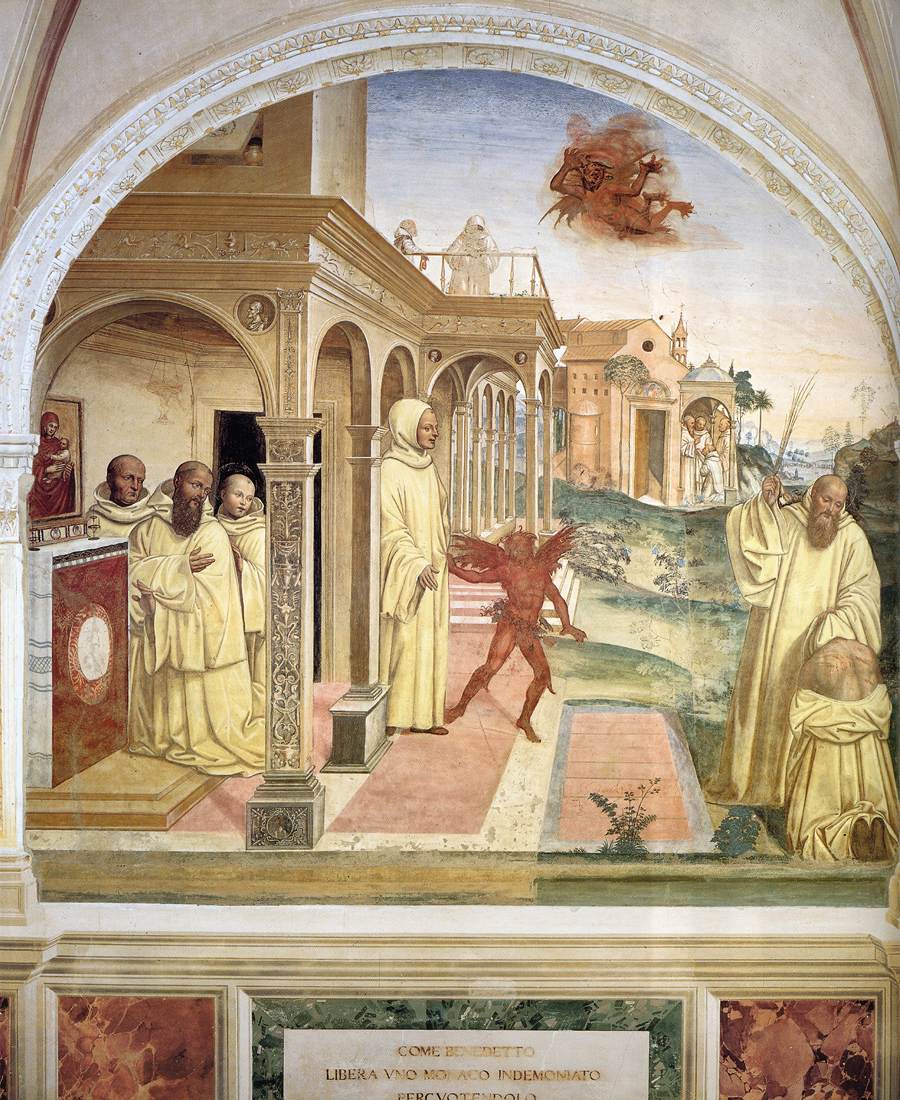The painting appears to be an ancient religious artwork possibly found in a Catholic cathedral. Dominated by intricate columns and white buildings, the scene is set within an arched structure. At the bottom of the image, partially cut-off Latin text reads: "come end it to Libra... Monaco in Dominique". The painting depicts a gathering of around eleven figures, predominantly men in beige or off-white robes, engaged in prayer or religious activities. A significant portion of the scene features a mother-like figure clothed in red on the left and a bearded religious figure holding a staff on the right. At the image's center is a striking red-winged figure, probably a demon, indicating punishment, surrounded by a red cloud. Two smaller devil-like creatures seem to lead the figures unwittingly. The background includes a blue sky melded with white hues, green and yellow grass, red and white marbled stairs, and a balcony with two onlookers. The entire composition gives a sense of both worship and underlying sinister influence, reinforced by the red demonic presences.